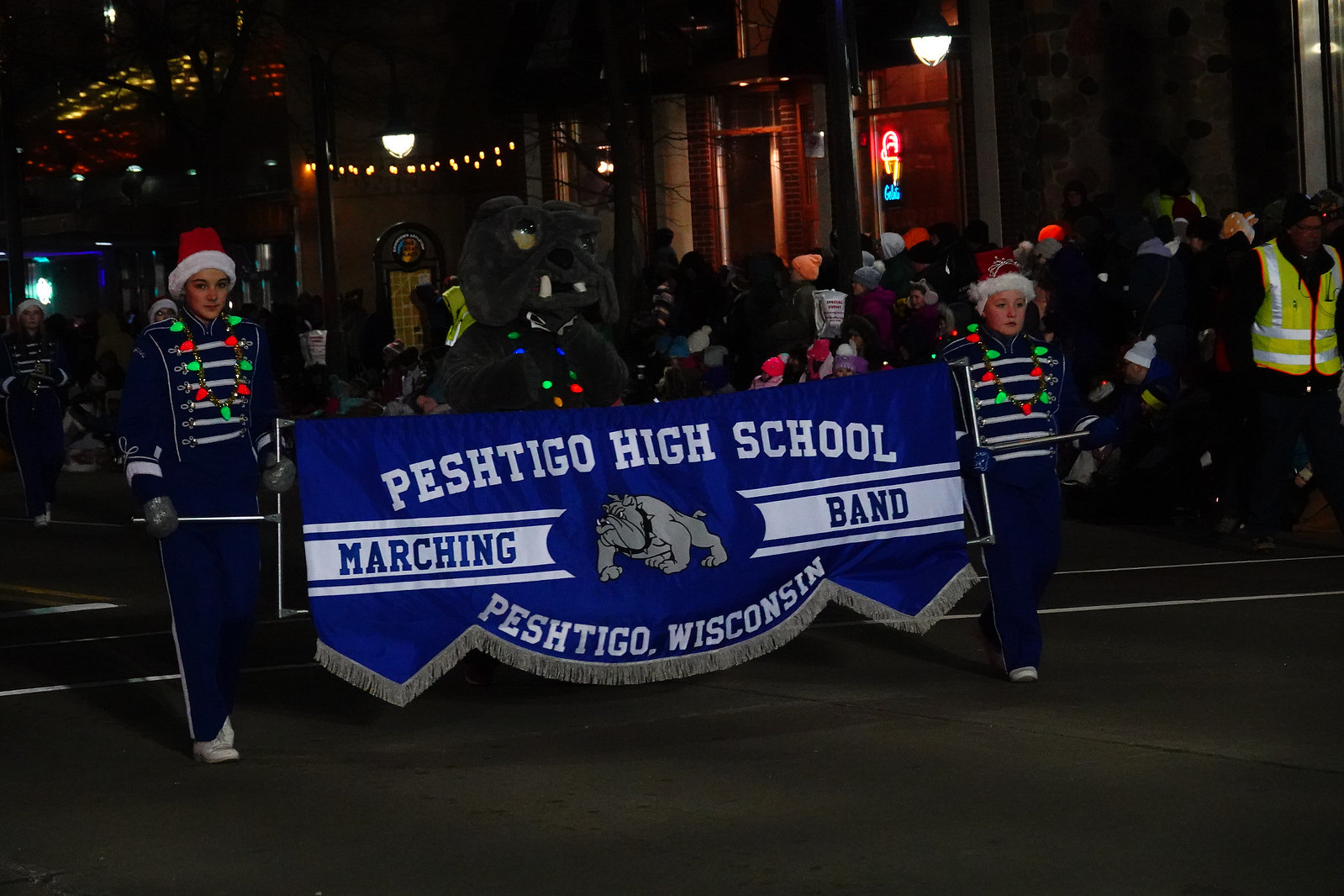In the dimly lit night, a festive Christmas parade winds through the streets, lined with excited onlookers and children. The central focus is the Peshtigo High School Marching Band, prominently displayed as two young women, dressed in blue and white uniforms with white stripes, hold a large blue and white banner that reads "Peshtigo High School Marching Band, Peshtigo, Wisconsin," adorned with a gray frill at the bottom. They each wear Santa hats and are illuminated by green and red Christmas lights draped around their necks. Striding behind them is a mascot, a person dressed as a gray bulldog decorated with vibrant Christmas lights. The streets are bustling with observers, some of whom are standing next to police officers, all gathered to enjoy the lively parade that captures the spirit of the Christmas season. String lights twinkle in the background, adding to the enchanting holiday ambiance of this night-time celebration.